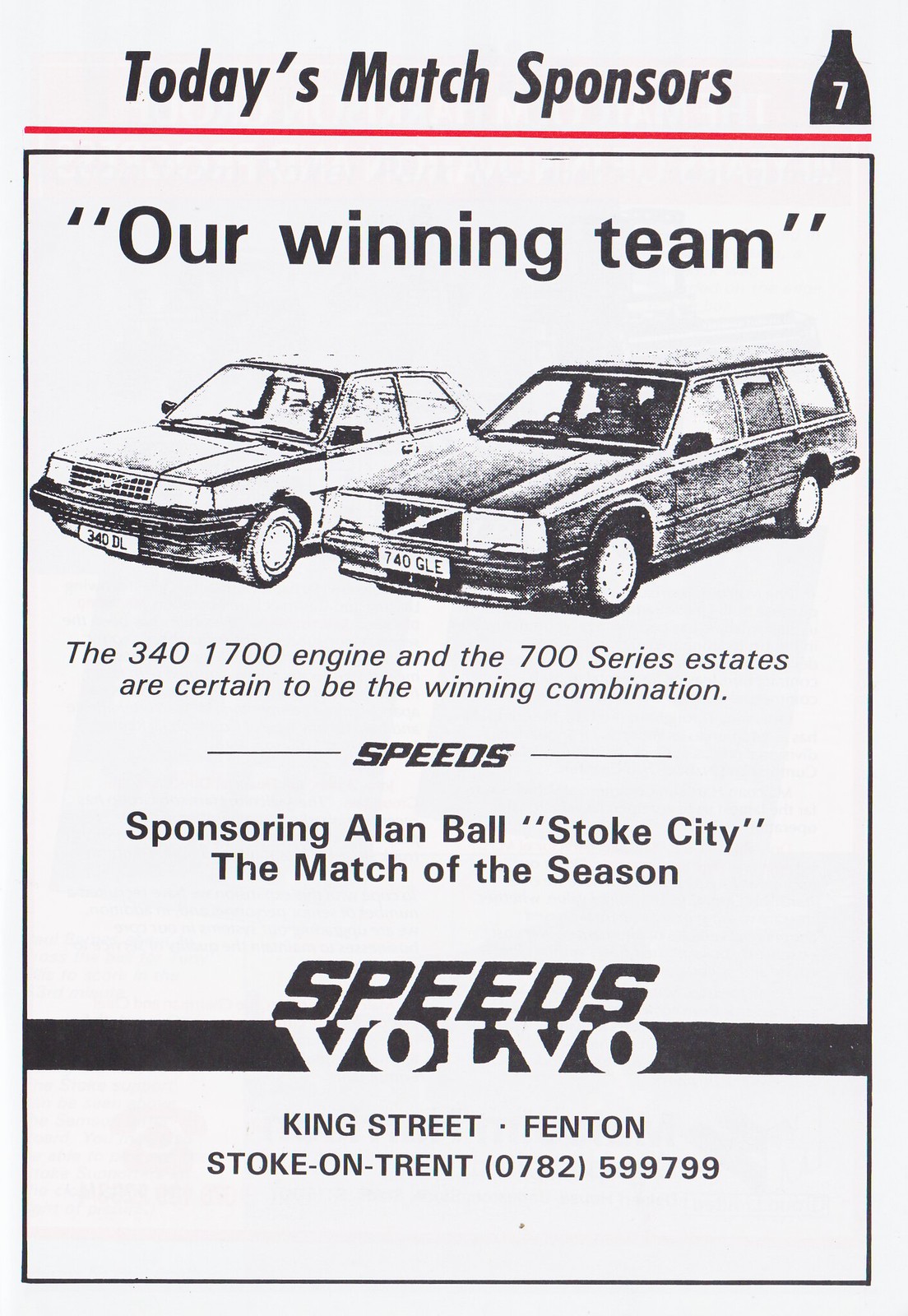The image is a black-and-white scanned flyer or pamphlet advertising Volvo cars, prominently featuring the headline "Today's Match Sponsors" at the top. It highlights the number 7 on a black, bottle-shaped logo and declares "Our Winning Team." The central focus of the advertisement includes two Volvo vehicles, a station wagon and a regular car. The vehicles are identified as the 340 with a 1700 engine and the 700 series estates, portrayed as a winning combination. Additionally, it reads "Speeds sponsoring Allen Ball, Stoke City, the match of the season." At the bottom, the flyer provides the dealership's details: "Speeds Volvo, King Street, Fenton, Stoke-on-Trent, 0782599799." The image underscores the association between the car models and the event, suggesting a strong, winning partnership.